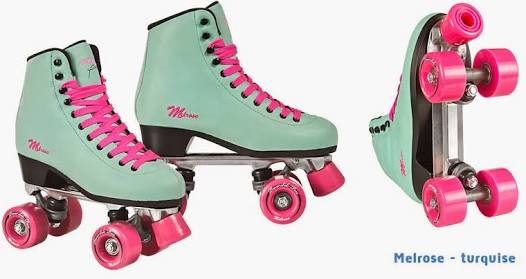This image appears to be a product advertisement on a white background, featuring three views of the same roller skate model. The skates are predominantly white with a feminine design, showcasing various bright pink accents such as the laces, wheels, front stopper, and a logo on the side in script. The footwear sports a small, approximately one-inch black heel mounted on a metal frame that connects to four vibrant pink wheels and a pink stopper at the front for braking.

In the photo, the skates are arranged to give a comprehensive view: the left skate is tilted to display the front, the middle skate provides a clear side profile, and the right skate is flipped to show the underside, highlighting the roller's full structure and wheel placement. In the bottom right corner of the image, "Melrose-Turquise" is written in blue text, with a notable misspelling, as "turquoise" should be "T-U-R-Q-U-O-I-S-E." The overall composition emphasizes the skate's vivid color scheme and stylish appeal.